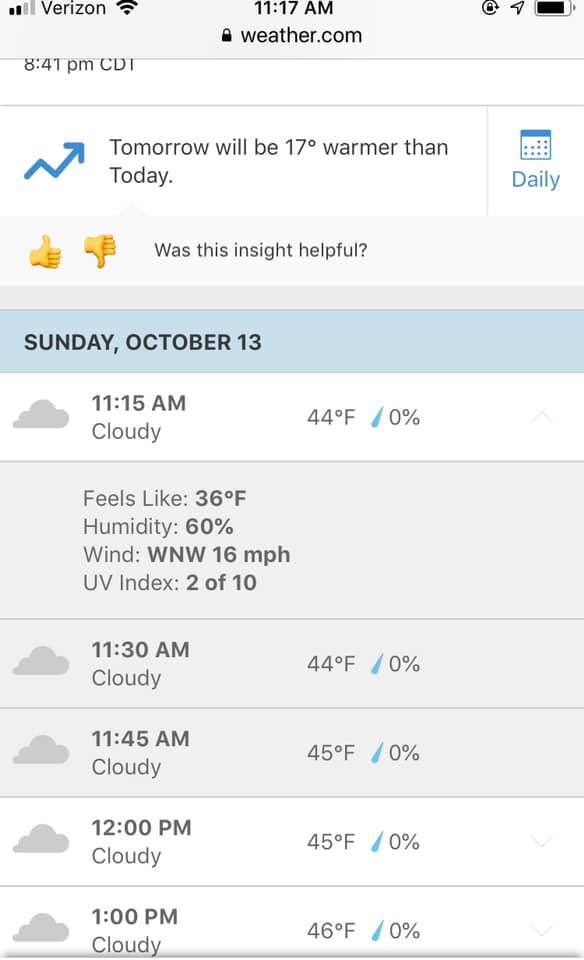The image is a phone screenshot, likely from an Android device, with the cellular network displaying Verizon at the top. The status bar on the upper-left shows two highlighted signal bars out of four, indicating partial reception, followed by the Wi-Fi icon. In the center of the status bar, the current time is shown as 11:17 a.m. On the right side, there are additional icons including a send icon (an arrow pointing up and to the right) and a battery icon. This upper section appears to be partially cut off, leading into a light gray banner that displays "8:41 p.m. CD", with the "T" seemingly cut off, implying "CDT".

Below the gray banner, a message is displayed with an upwards arrow symbol and text reading "Tomorrow will be 17 degrees warmer than today". Next to this message, on the right side, a calendar icon is visible with the word "Daily" underneath.

Underneath this section, there is another gray banner featuring thumbs up and thumbs down icons alongside the text "Was this insight helpful?" Below this, a small gray area transitions into a light blue banner that reads "Sunday, October 13th, 11:15 a.m. Cloudy, 36 degrees."

Continuing down, the hourly forecast is provided:
- "11:30 a.m. Cloudy"
- "11:45 a.m. Cloudy"
- "12:00 p.m. Cloudy"
- "1:00 p.m. Cloudy"

The temperatures for each time increment are displayed, starting from 44 degrees and ending at 46 degrees. Each time slot is accompanied by a small gray cloud icon on the left, signifying the cloudy weather conditions throughout.